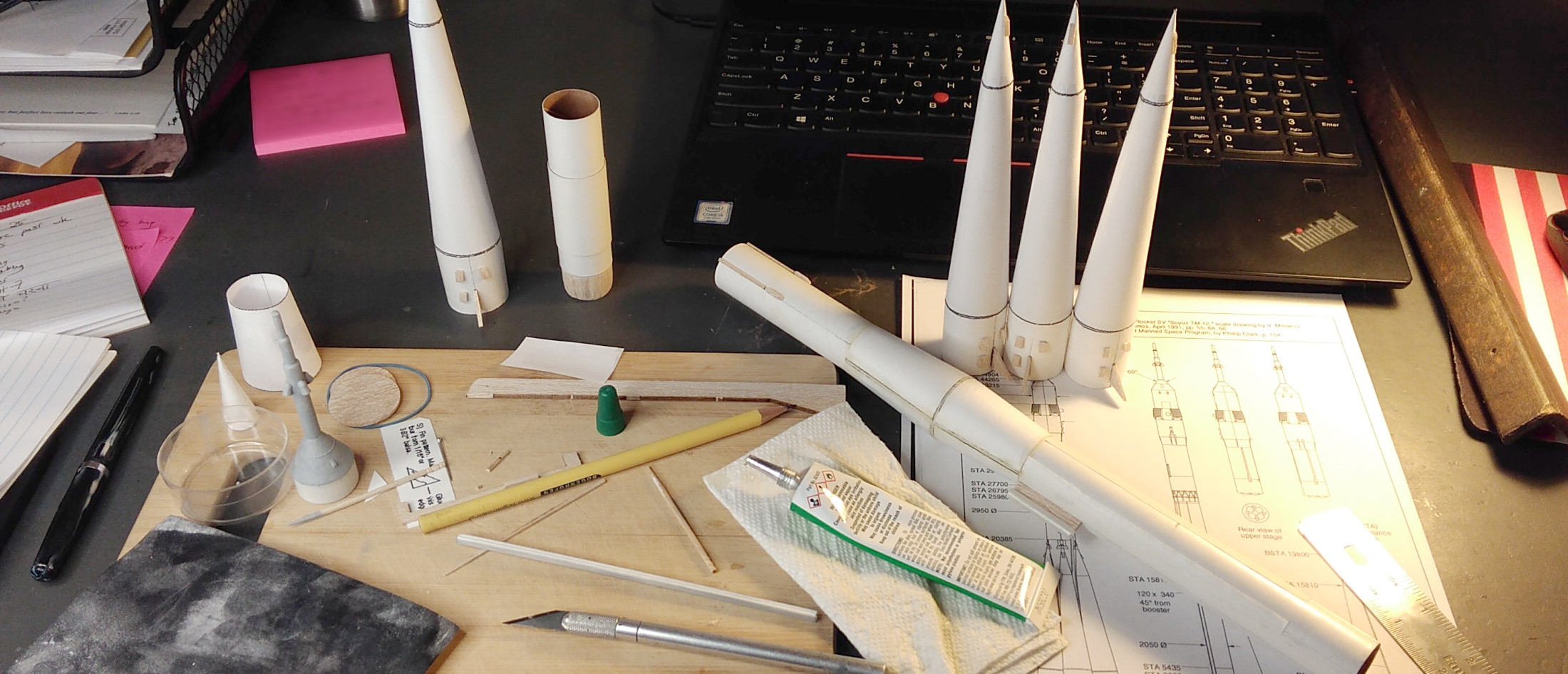The photograph depicts an indoor workspace, likely a hobby station dedicated to model rocket construction. Prominently featured in the background is a black laptop, serving as a focal point alongside a paper stacker filled with papers and hot pink Post-It notes. The desk is cluttered with a variety of crafting tools including an X-Acto knife, pencils, tubes of glue, sandpaper, and dropper bottles, all situated on a cutting board. Spread out in front are instructions showing detailed diagrams of the rocket being assembled. The model rocket components, including three to four pointed top sections and one long central body piece, are laid out meticulously. These components, appearing to be constructed from paper, suggest that the model is purely decorative. The detailed and busy arrangement illustrates a project in progress, capturing the intricate process of building a model rocket.